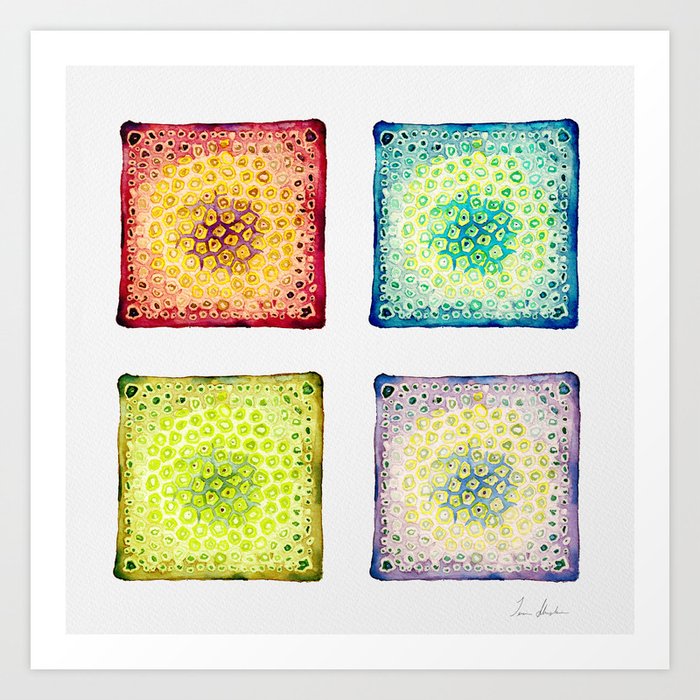This image features a framed piece of art hanging on a light gray wall. The artwork itself is encased in a white border, with an interior background of very light gray, featuring a textured look. The composition consists of four distinct colored squares arranged to form a quadrant with white spacing in between. The top left square is a red-pink hue adorned with yellow circular patterns. The top right square is navy blue with intricate designs in yellow and green. The bottom left square offers a yellowish-green tone with neon green patterns, while the bottom right showcases shades of light and dark purple with yellow motifs. Each square has darker accents at its center and is decorated with circular shapes that have small black dots in the middle, resembling intricate patterns or textures. A signature in black script is visible on the lower right corner of the artwork.